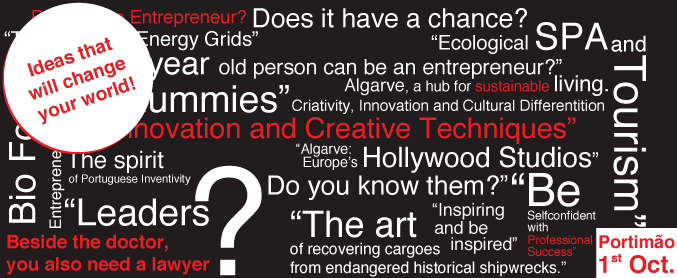This advertisement poster, designed for an event held in Puerto Mayo on October 1st, features a striking black background with various phrases in white and red text, creating a canopy of ideas. At the top left corner, a white circle contains red text that proclaims, "Ideas that will change your world!" Surrounding this circle, the poster is densely packed with diverse and somewhat eclectic phrases, ranging from "Does it have a chance" and "Ecological SPA" to "Innovation and creative techniques" and "Hollywood studios."

The poster's wide design, double in width compared to its height, allows for an expansive display of words. In the middle and along the right side, it highlights concepts such as "Entrepreneur," "Energy grids," "Tourism," "Algarve: A hub for sustainable living," and "Creativity, innovation, and cultural differentiation." It also features thought-provoking statements like "The spirit of Portuguese inventivity," and questions such as "Leaders?" and "Do you know them?"

Additional intriguing lines include "Besides the doctor you also need a lawyer," "Be self-confident with professional success," and "Inspiring and be inspired." Among these phrases is a curious mention of "The art of recovering cargoes from endangered historical shipwrecks," adding a sense of mystery and historical depth. The visually engaging combination of colors and words aims to captivate and provoke thought, offering a glimpse into the diverse topics the event promises to cover.